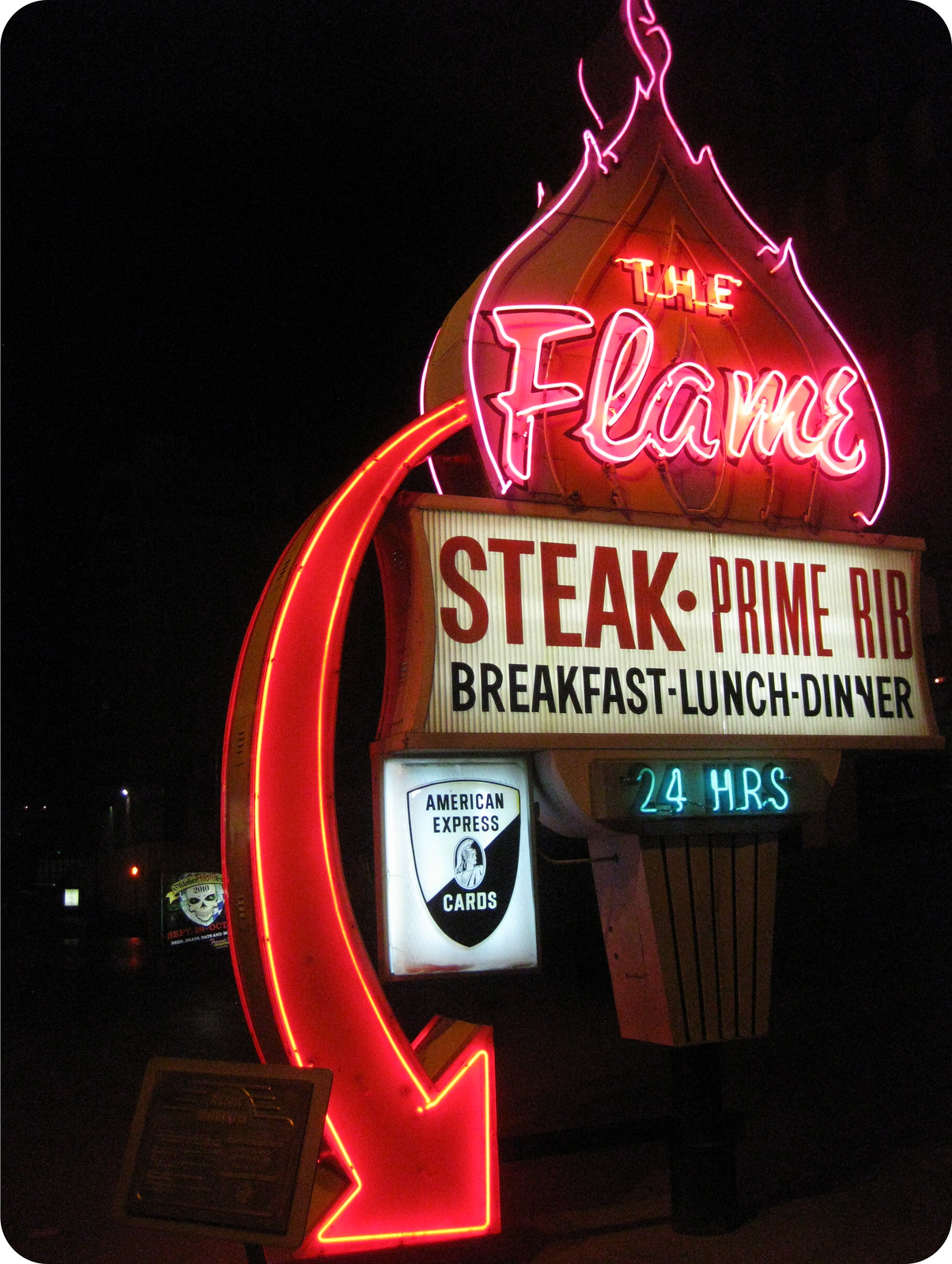This nighttime photograph captures an intricately detailed neon sign for "The Flame," a restaurant once renowned in Las Vegas. The central element is a vibrant red neon outline shaped like flames, encasing the restaurant's name, "The Flame," written in bold, cursive bubble text. Below this striking centerpiece is a backlit sign listing the restaurant's offerings: "Steak, Prime Rib, Breakfast, Lunch, Dinner," in black lettering. To the right, a small blue neon sign announces the restaurant's round-the-clock service with "24 Hours," while a black and white sign advertises that American Express cards are accepted. A curving neon arrow descends from the flame, directing potential patrons toward the restaurant. The photograph evokes a sense of nostalgia, hinting at the historic allure of this once-famous Las Vegas dining spot.